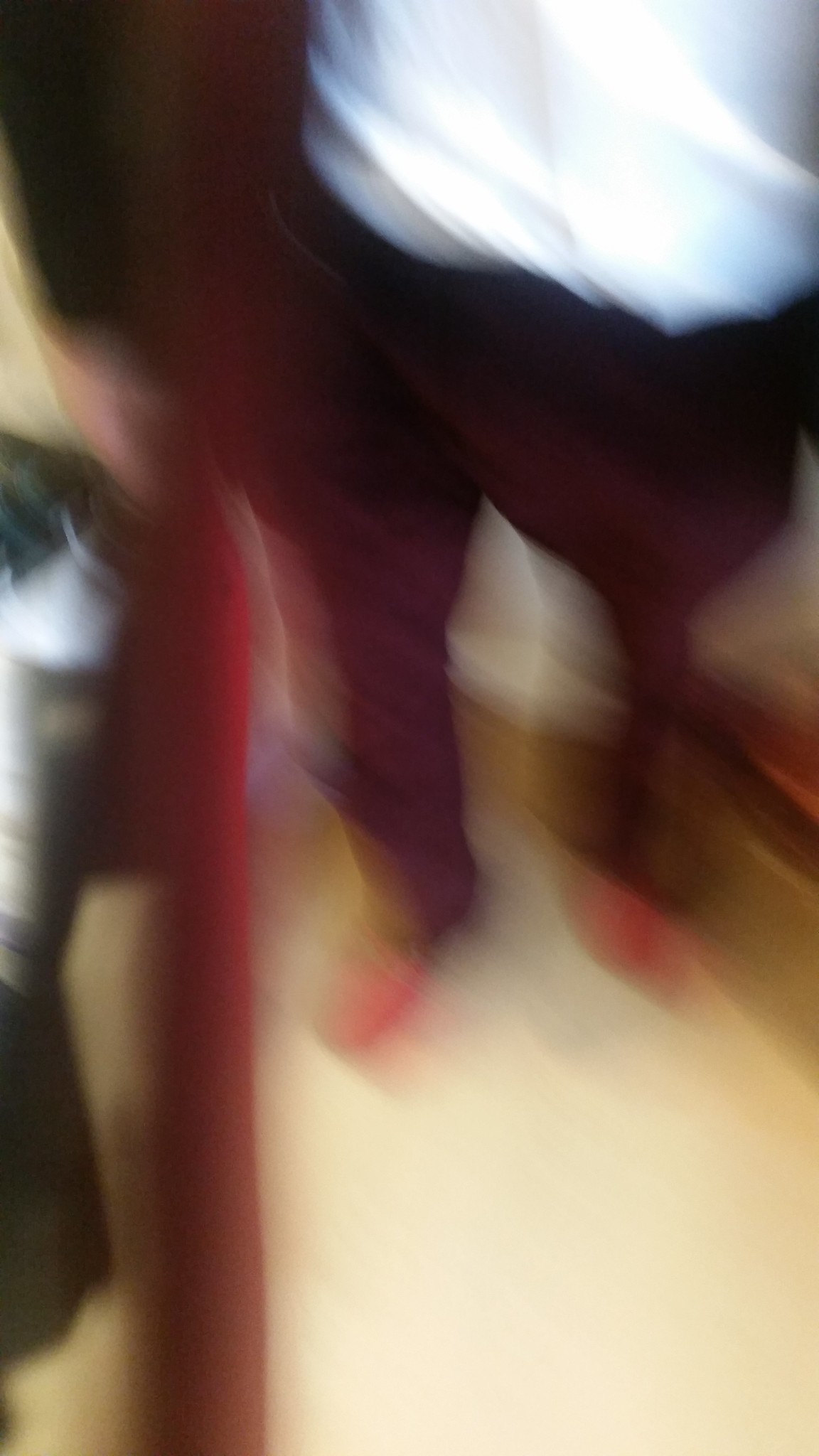This very blurry photograph, likely taken in portrait mode inside a building, captures a man from just below chest height down to his feet. He stands on a plain, beige tile floor. The man is dressed in dark maroon-colored pants with a matching suit jacket over a white button-down shirt. His footwear appears red, which could be either shoes or socks, though the blurriness makes it difficult to discern. His right hand rests by his side. Along the left edge of the image, there is something red and fuzzy, possibly part of a chair, with a black and white patterned section. Additionally, a dark figure with a white design on their front is barely visible at the far left.